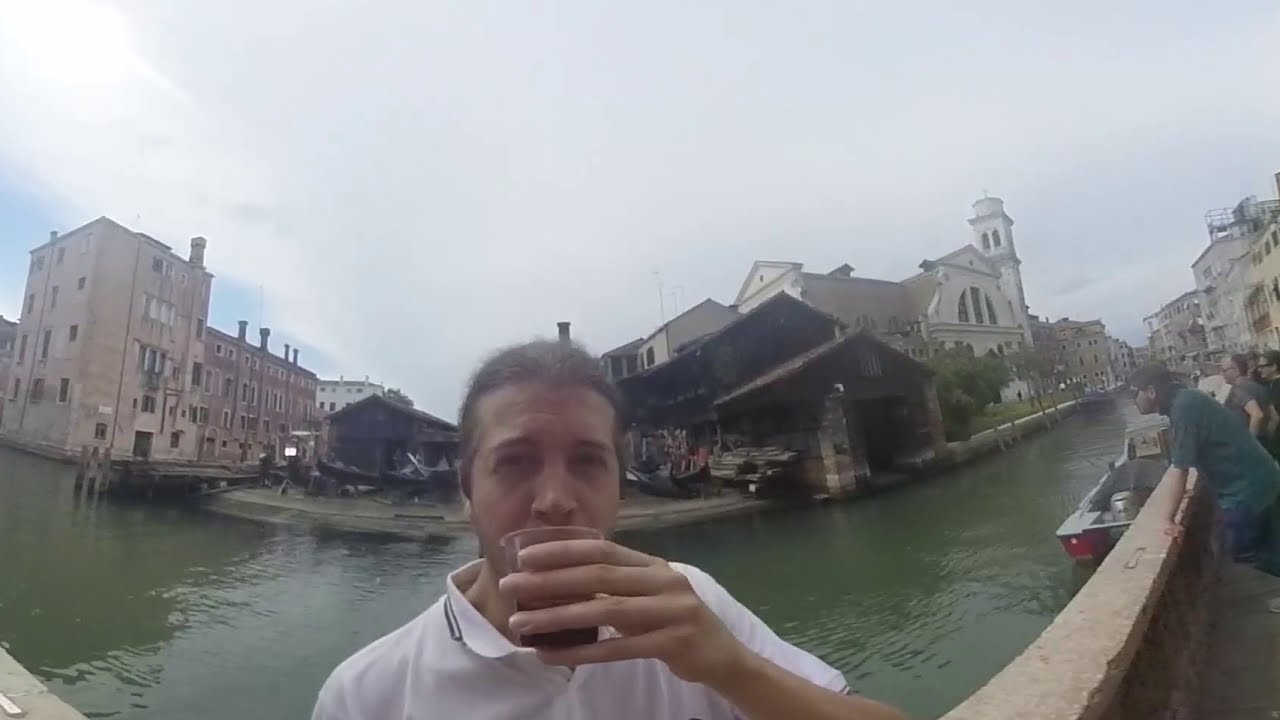The photograph captures a young man with dark skin, wearing a white shirt, drinking a beverage from a clear plastic cup near a canal in an urban environment. His hair is pulled back into a ponytail. The scene is somewhat misty and overcast, giving the image a slightly blurred, yet atmospheric quality. Behind him, water flows through the city, bordered by a stone breakwater on which several people are leaning, gazing out at the water. Some of these onlookers wear sunglasses despite the cloudy weather. In the background, a mixture of three- to four-story buildings line the canal, dominated by a large church, indicative of a European city. Boats are docked along the canal, adding to the busy yet serene scene. The water in the canal has a greenish tint, possibly from algae or reflections.